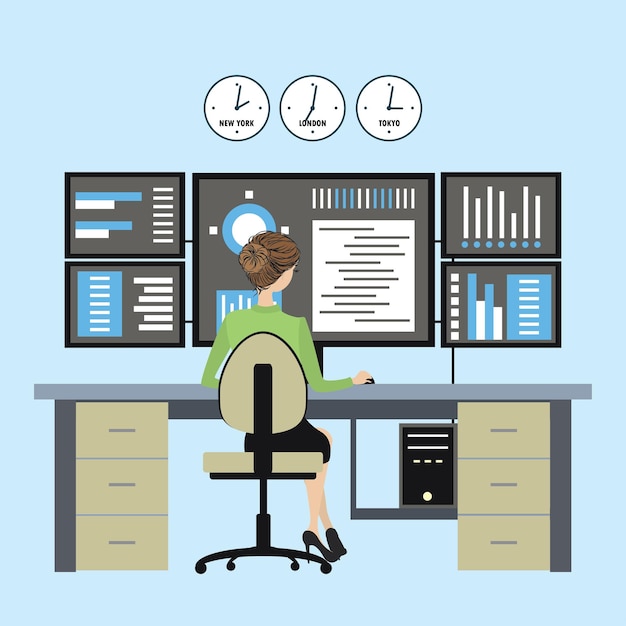In this detailed animation frame or rendering, a woman is depicted sitting at her desk. She appears to have blondish-brown hair neatly styled in a bun. Her complexion is light, and her black eyelashes provide a subtle yet elegant touch to her facial features. Notably, she is not wearing glasses.

Her attire consists of a green long-sleeve top paired with a slim-fitting black skirt. Completing her outfit are black high-heeled shoes. She sits comfortably on a chair featuring a yellowish-beige cushion, backed by a black frame equipped with black wheels for mobility.

The desk she occupies is organized and functional, boasting six yellowish-beige drawers accentuated with gray lines that serve as handles. The surface of the desk is predominantly gray. Positioned prominently in front of her is a large computer monitor, flanked by two smaller monitors on each side, all connected in parallel, allowing for an expansive, multiscreen workspace.

Additionally, the scene includes three clocks on the desk, each indicating different time zones. They are carefully labeled "New York," "London," and "Tokyo," suggesting that she may be involved in an international business or project.